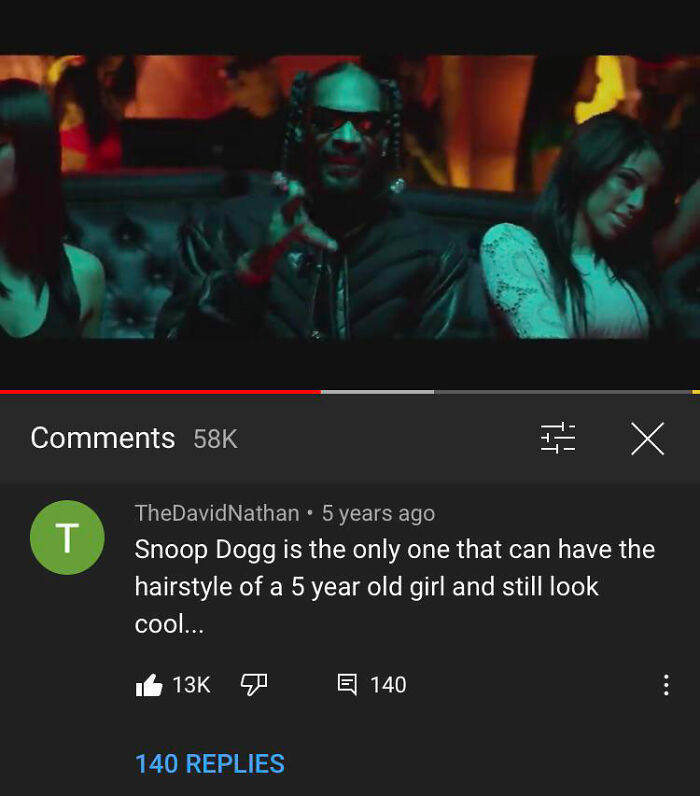The image captures a screenshot of a YouTube video featuring Snoop Dogg, along with a glimpse of the comment section. The video itself is framed by horizontal black bars at the top and bottom, indicating that it is currently playing. 

In the foreground, Snoop Dogg is prominently seated on a sleek, black leather couch. He sports black glasses with a faint red reflection and is clad in a thick, puffy black jacket. His signature dreadlocks hang down on either side of his head. Surrounding him are two elegant women: the one on his left has shoulder-length, straight black hair and is dressed in a sleeveless black outfit, while the woman on his right, with olive-toned skin, has black hair and wears a long-sleeved white lace dress. The background is filled with a reddish-orange hue and some individuals are seen milling about, adding to the lively atmosphere.

Beneath the video, the comment section is set against a dark gray background. At the top, it indicates there are 58k comments. The visible comment is from a user named David Nathan, posted five years ago, which humorously states, "Snoop Dogg is the only one that can have the hairstyle of a five-year-old girl and still look cool." This comment has garnered 13,000 likes and 140 replies.